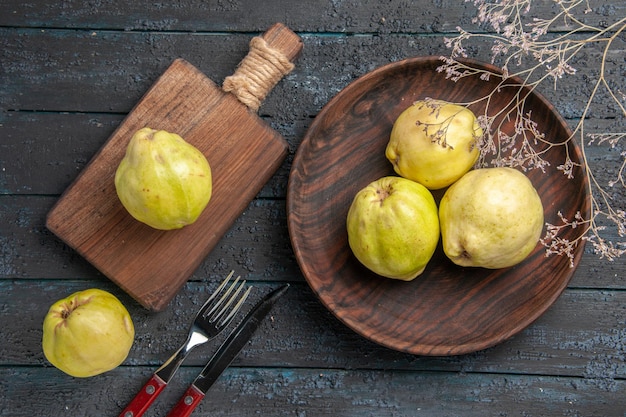This top-down, realistically captured photograph showcases a rustic kitchen scene set on a dark, rough, grayish wooden table. In the bottom left, there’s a knife and a fork with red wooden handles and stainless steel blades and prongs. Adjacent to the utensils, on the left, sits a wooden cutting board with a piece of greenish-yellow, gourd-like fruit on it. Another similar fruit is partially placed on the table, leaning against the cutting board that features a wooden handle wrapped in rope. Next to the cutting board is a shallow, plate-like wooden bowl holding three more greenish-yellow, gourd-like fruits. In the top right corner, delicate sprigs of a plant with light brown stems and tiny purple flower buds add a touch of natural elegance to the setting. The meticulous arrangement and the earthy tones of the wooden elements and fruits blend together, evoking a sense of rustic simplicity.